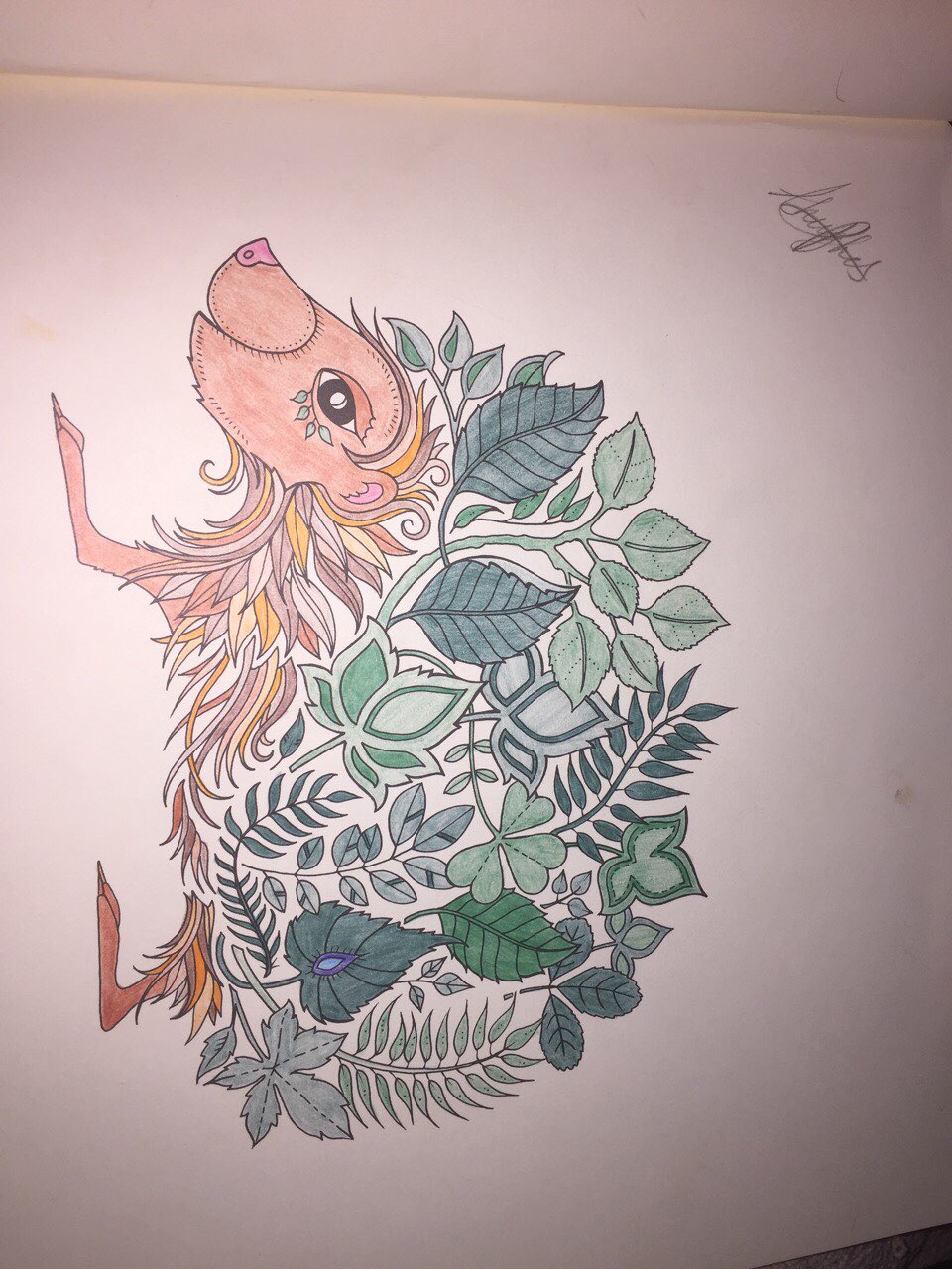The image features a detailed and artistically crafted sketch of a hedgehog, drawn on a piece of white paper about the size of standard printer paper. The sketchbook page is oriented vertically, but the hedgehog is designed to be viewed horizontally. This whimsical, cartoony-styled hedgehog is composed entirely of earthy elements. Its charming face is pale pink with a nose that appears stitched on and large, expressive brown eyes adorned with leaf-like tattoos beneath them. The body of the hedgehog is a blend of various shades of brown, crafted from an intricate array of leaves and ferns in place of traditional spikes. These leaves, ranging from maple to oak, and big long ferns, are colored in diverse shades from dark to light forest green, contributing to the overall colorful and vibrant feel of the artwork. A small section of the image also reveals what appears to be a crossed-out name or word in the upper right corner. The background is light-colored, possibly the surface of a table or white wall, providing a contrasting backdrop that emphasizes the beauty and detail of this carefully colored-in, plant-inspired hedgehog.